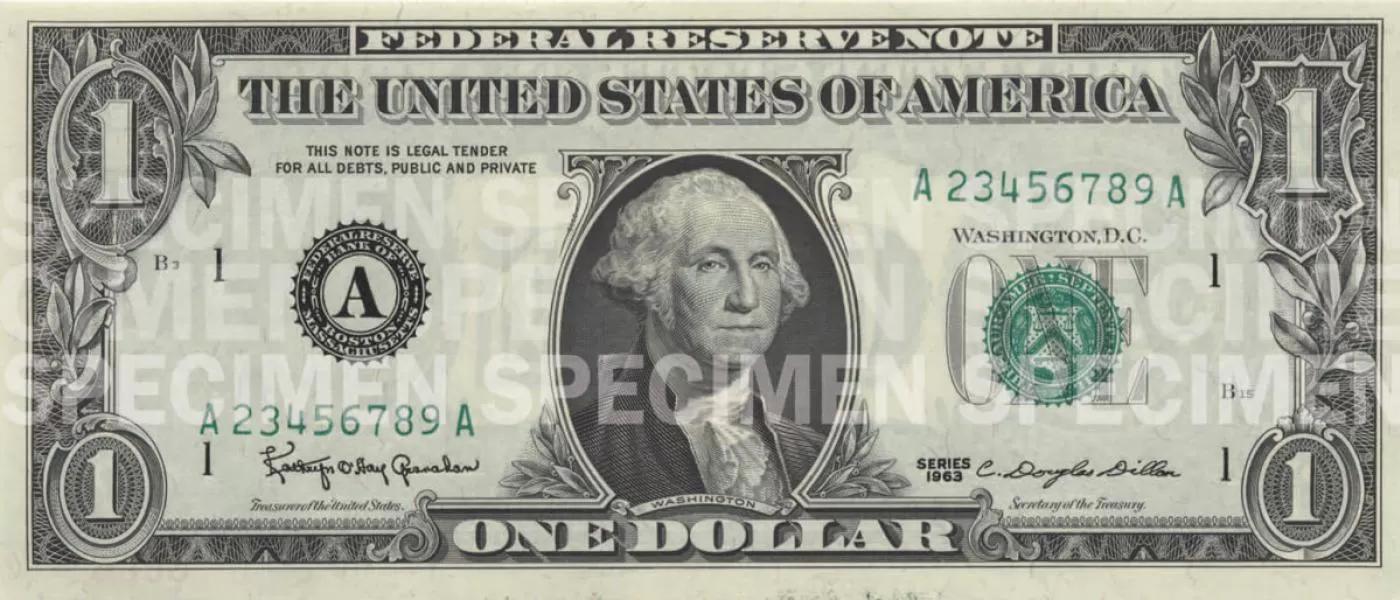Photograph of a U.S. one-dollar bill displayed against a plain white background. The bill is clearly identified as a specimen, with three bold, white "SPECIMEN" labels prominently overlaid across its surface, making it unmistakably non-circulable. At the top of the bill, the text "Federal Reserve Note" and "The United States of America" are visible. Serial numbers are present, along with the number "1" in each corner. The center of the bill features an image of George Washington, and the signatures of the Secretary of the Treasury and the Treasurer of the United States are also seen. Besides the "SPECIMEN" markings, the bill appears to be a standard U.S. one-dollar note.